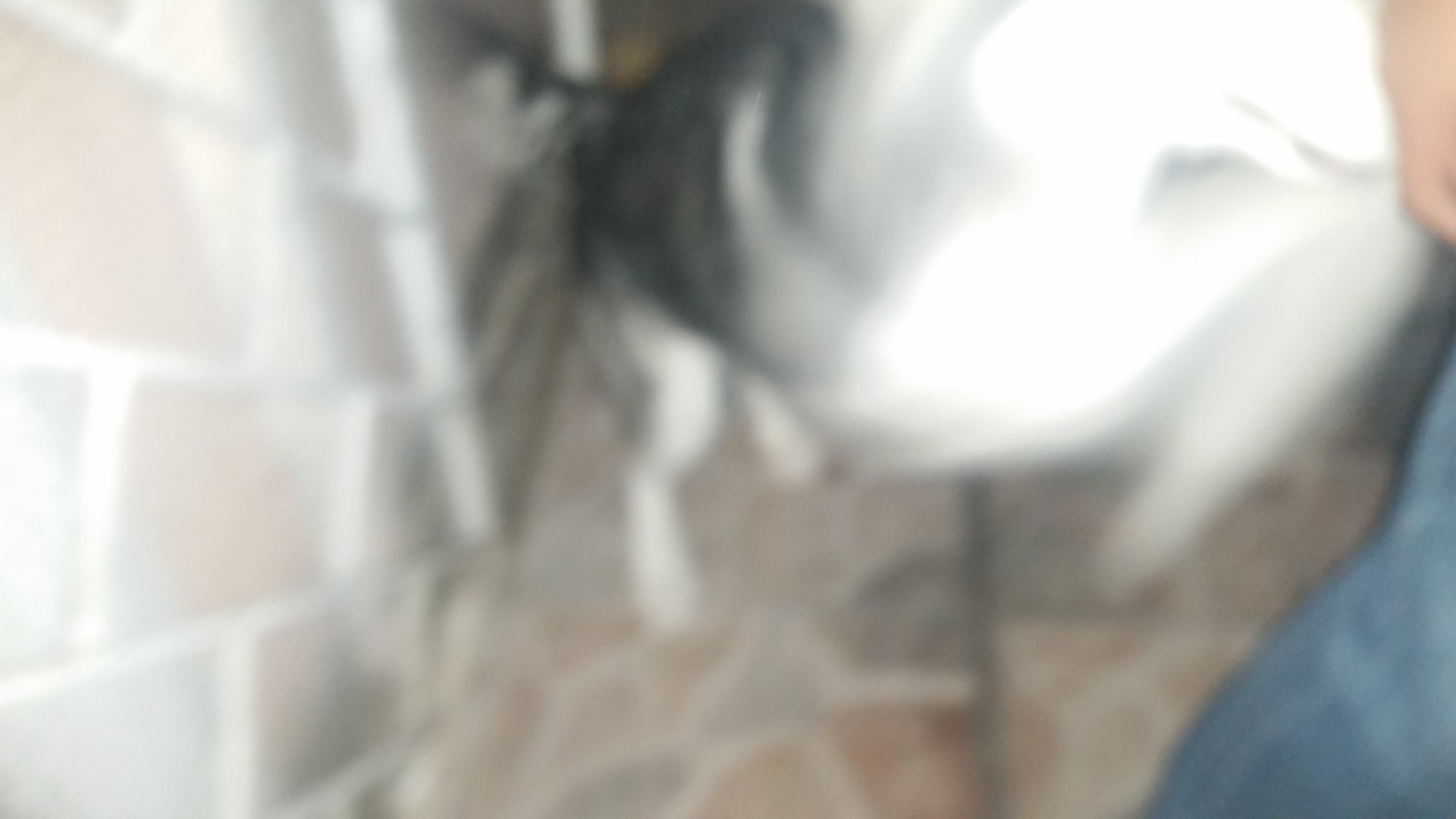A slightly blurry image featuring a husky dog, primarily white with darker shading along its back, tail, and legs. The dog appears to be standing on its hind legs on a stone surface characterized by a mix of gray and red, creating a faded mosaic effect. To the top right, a human hand is visible along with the side of someone's jeans, suggesting interaction with the dog. The background includes a similarly colored wall, against which the husky's back and tail are positioned. Despite the blur, the playful stance of the dog amidst the muted-toned stone and wall surfaces is evident.